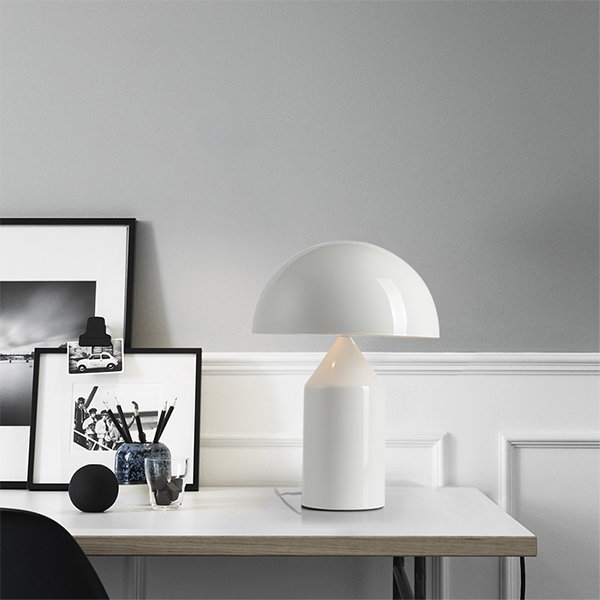The color photograph showcases a meticulously arranged living room or study with a prominent white wood desk positioned against a medium gray wall featuring white wainscoting. The desk's centerpiece is a glossy, dome-shaped, white table lamp made from either ceramic or plastic, which is lit. To the left of the lamp, a pair of black-framed, black and white photos rest against the wall, one prominently depicting a scene with people walking down stairs and another featuring a landscape. A picture of a European car, attached with a clasp, can be seen clipped to one of the frames. Adding to the desk's decorative elements, there is a glass jar filled with paintbrushes and another tumbler holding small black cubes. Situated to the lower left corner is the visible part of a black office chair. A small round device, likely an Echo Dot, also sits on the desk. The careful arrangement of these objects against the minimalistic backdrop creates an elegant and organized aesthetic.